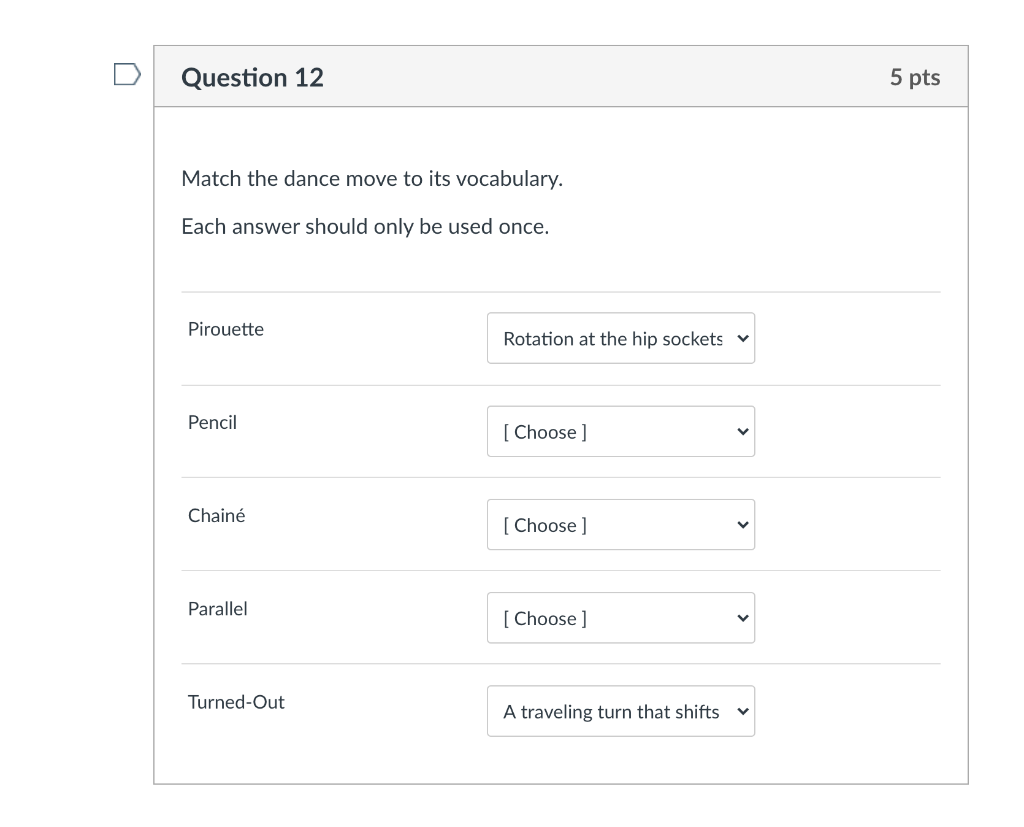The image showcases a section of a digital menu or online questionnaire, specifically featuring "Question 12" at the top. On the left-hand side, there is a highlighted rectangular box containing a white arrow symbol, pointing downward, which indicates a dropdown menu for selection. Within the same highlighted box, on the right-hand side, the text "5 points" is displayed.

Beneath this main section, there is an instruction that reads, "Match the dance move to its vocabulary. Each answer should only be used once." 

In the left-hand column, the dance term "Pirouette" is spelled out as "P-I-R-O-E-T" and corrected to "P-I-R-O-E-T-T-E". Adjacent to this term, in the dropdown box below, it states "Rotation at the hip sockets."

Further down, the form lists different dance terms with corresponding dropdown boxes:

- "Pencil" with a dropdown menu labeled "Choose".
- "Chainé" (spelled as "C-H-A-I-N-E" with an accent) also with a "Choose" dropdown.
- "Parallel" with another dropdown box labeled "Choose".
- "Turn out" described as "a traveling turn that starts" in the selection box, followed by another dropdown menu.

The overall design of the form features a white background with black font, giving it a clean and straightforward look.